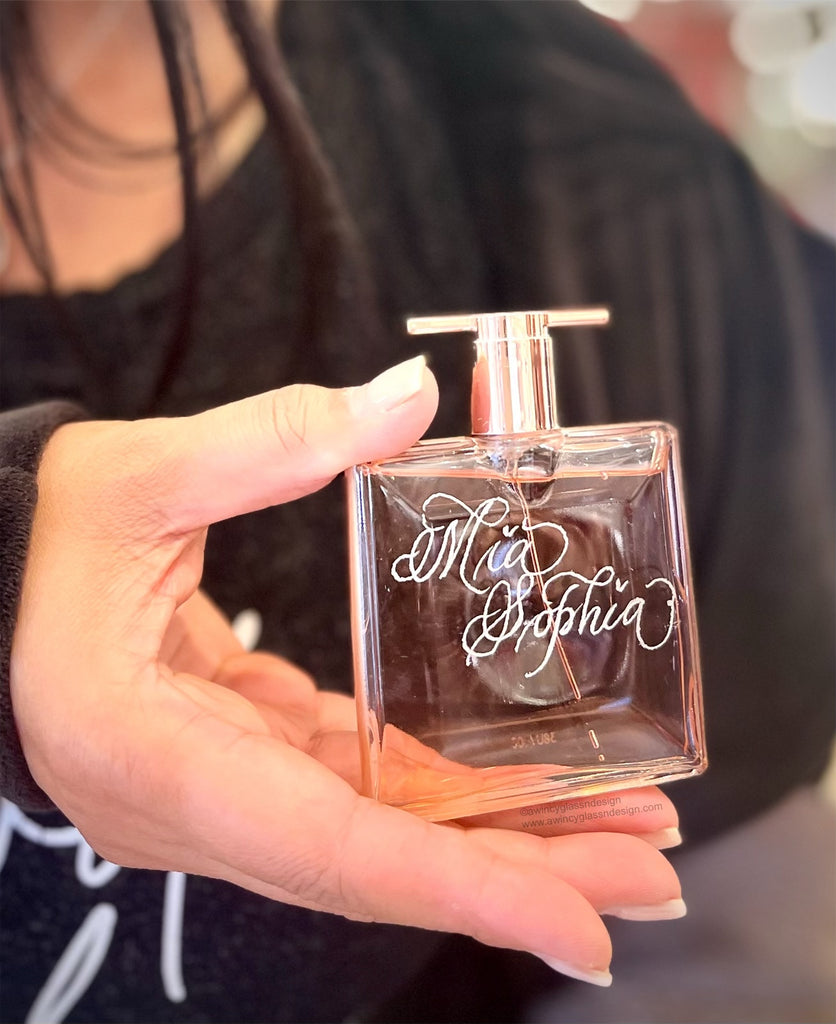The image showcases a close-up view of a woman's right hand delicately holding a square, clear perfume bottle that has a distinctive pink tint and a shiny, rose-colored metallic sprayer. The bottle is nearly filled to the top with pink-hued perfume. "Mia Sophia" is elegantly inscribed on the bottle in white cursive lettering. The woman, who has shoulder-length, dark brown hair cascading around her, is wearing a black long-sleeved shirt with indistinct white writing. Only her neck and partial chest are visible, effectively framing the focal point of the image—the perfume bottle. Her nails are natural with no polish, suggesting a light complexion. Additionally, faint text on the bottle reads "Wincey Glass and Design" with a website URL.